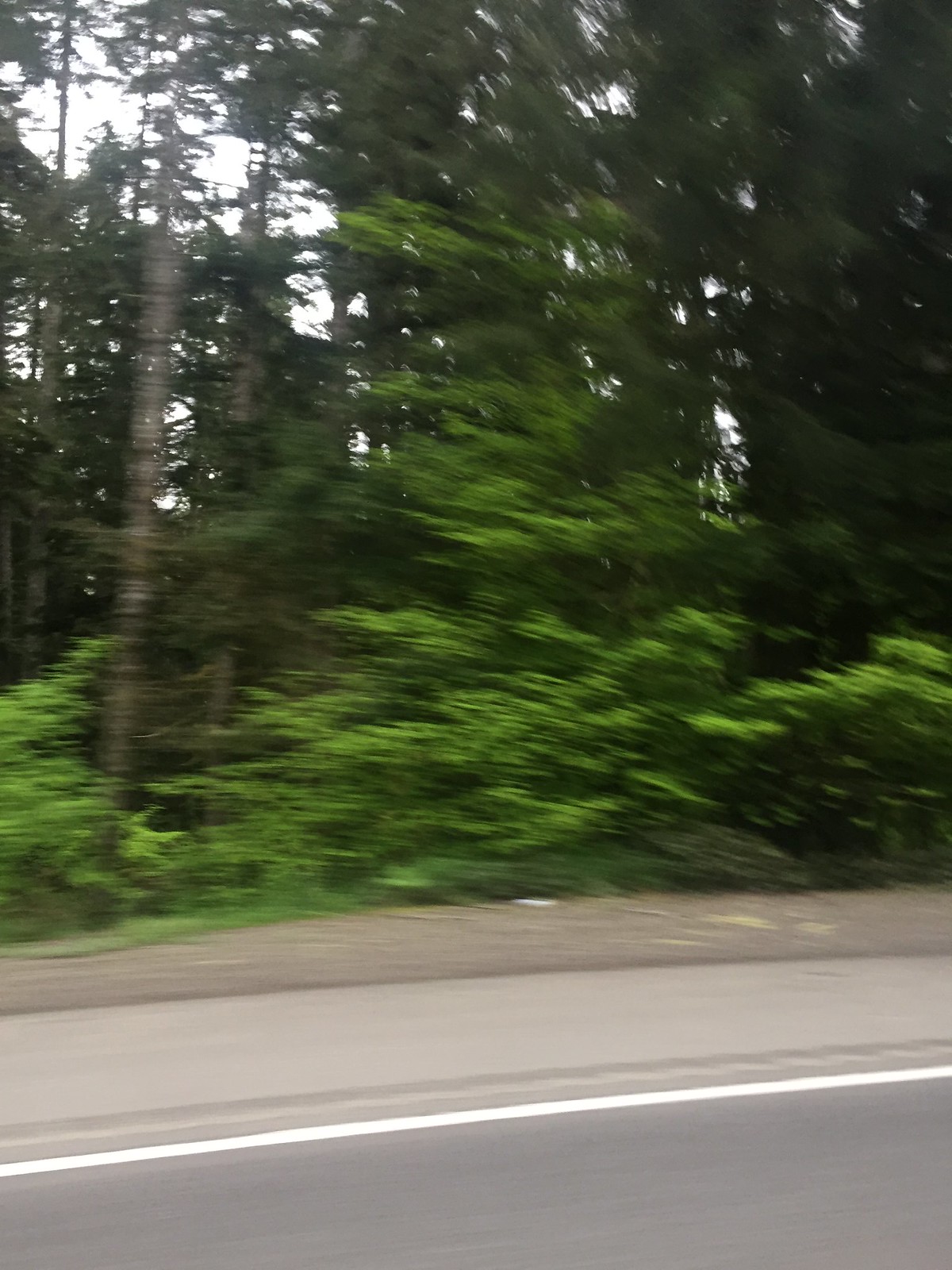This image captures the view from a moving car, taken through its window, resulting in noticeable motion blur. The foreground features the gray asphalt roadway with a solid white line along its edge, indicating the boundary of the blacktop. Beyond the road, there's a narrow shoulder and a stretch of light gravel or dirt. In the right-hand corner, the slope of the road is visible, enhancing the sense of movement. The background transitions into a dense forest, where tree trunks—some grayish and others brownish—are visible. The greenery varies, with some trees bearing light green leaves and others exhibiting a darker, hunter green hue, likely indicating a mix of deciduous and evergreen trees, such as firs or pines. You can also see areas with sparse foliage, revealing the forest floor. Light filters through the trees, suggesting an overcast sky that appears whitish-gray, contributing to the daytime setting of the image.